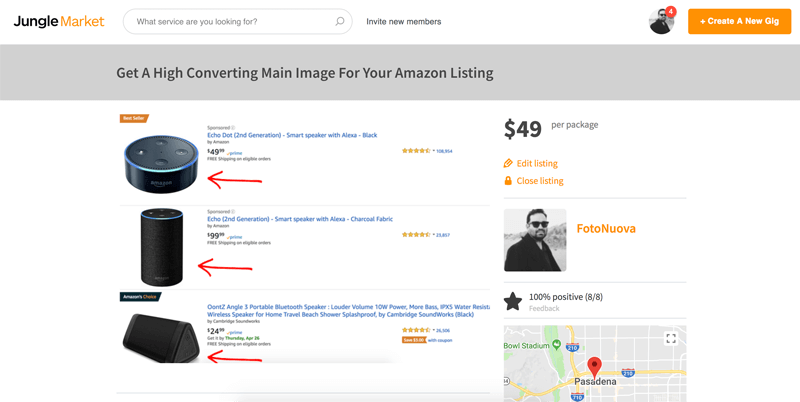The image is a screenshot from an online marketplace website called "Jungle Market," as indicated by the header at the top left corner. Beside the site name is a search bar with placeholder text reading "What service are you looking for?" On the right side of the header, there is an option labeled "Invite new members." 

Centrally displayed in the image is a prominent title that reads, "Get a high converting main image for your Amazon listing," suggesting a service being offered on the site. To the right of this title, the pricing for the service is clearly marked as "$49 per package."

Beneath this pricing information, two orange buttons are present labeled "Edit listing" and "Close listing," which likely provide options for managing the listing. 

Further down, the listing includes a photograph showing a man wearing sunglasses. To the right of his image, the text "Photo: New Alpha" is displayed, which might indicate the name of the image or the creator.